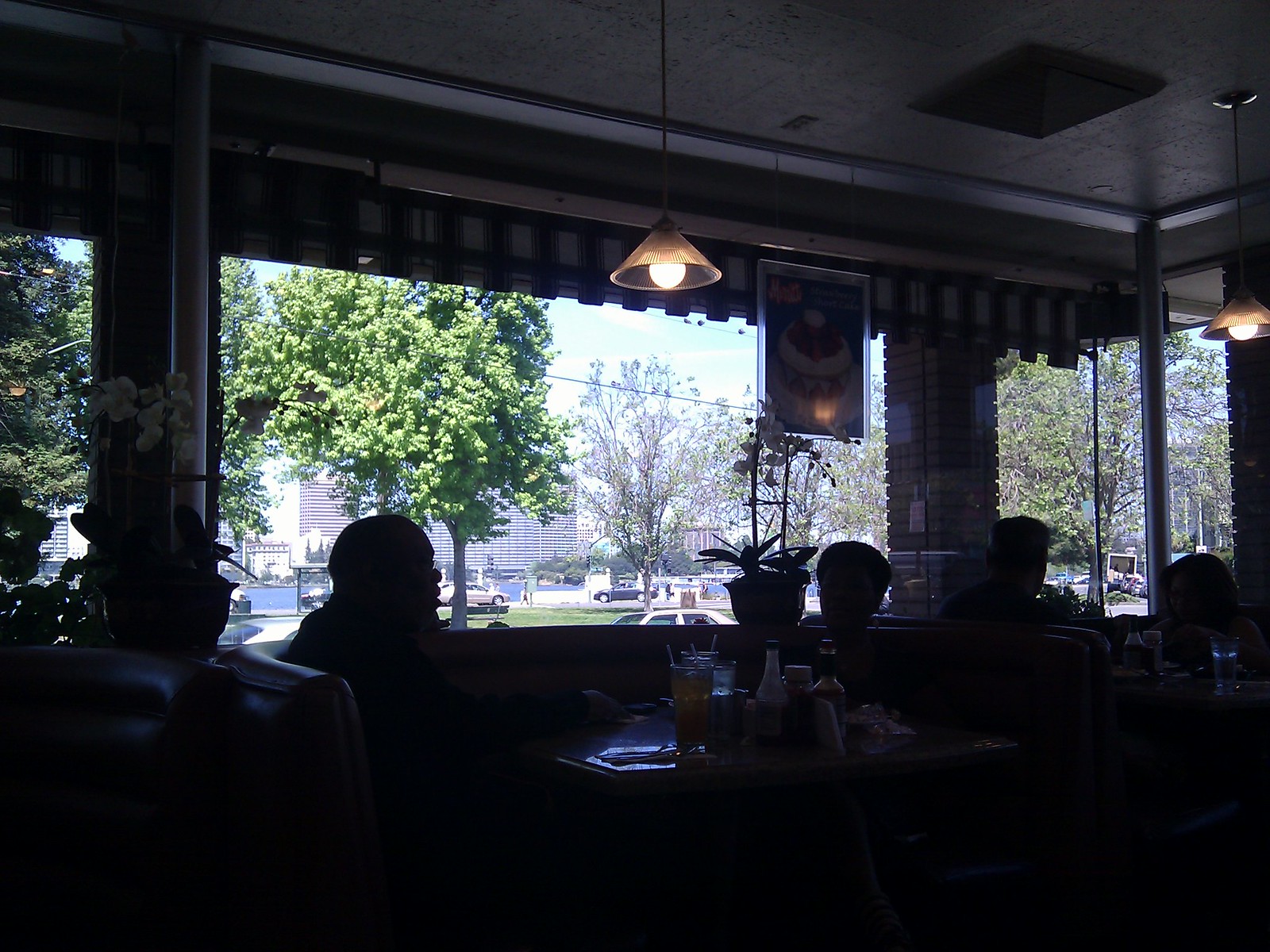In a dimly lit diner, the scene is shrouded in darkness with just a few golden chandeliers hanging from the ceiling, casting minimal light. The ceiling lamps are white with ornate golden fixtures, providing the only real illumination inside. Patrons are seated in booths, their faces obscured by the pervasive shadows. Three large rectangular windows offer a view of a bright daytime cityscape that contrasts starkly with the interior's gloom. Outside, there's a lush green tree with dense foliage, another tree that appears dead or barren, and distant semi-skyscrapers forming a part of the skyline. Several cars, including white and black ones, line what seems to be a road, and a blue river can be discerned beyond them. In the diner, two people are outlined in one booth, likely a man and a woman, with drinks visible on their table. A potted orchid rests on the windowsill, adding a touch of life to the otherwise dark setting. Beside them, another couple can be seen in a separate booth. The overall ambiance is a blend of dark interior with stark, bright outdoor elements, making for a striking contrast.